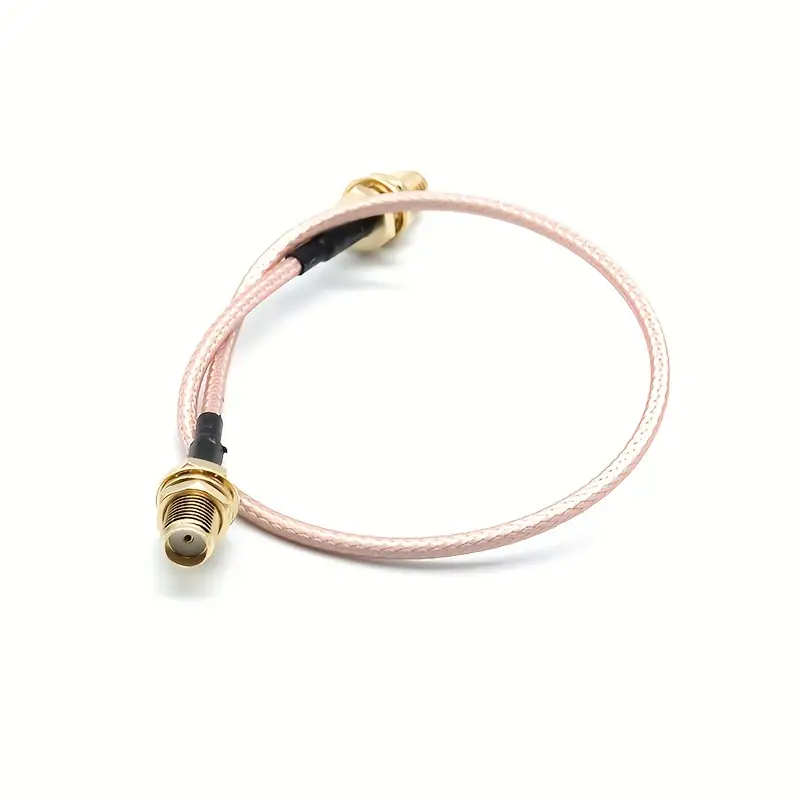This is a detailed product photo of a short, light pink or salmon-toned coaxial cable, approximately one to two feet in length. The cable features brass-colored coaxial connectors on both ends, secured by what appears to be black tape or heat-shrunk enclosures just before the connectors. The cable is neatly looped into a single circle for an artistic presentation, with the connectors positioned more toward the left side of the image. The ribbed texture of the cable and its looped form add an elegant touch, while the background is a plain white, emphasizing the product itself. The left-end connector is oriented towards the viewer, revealing a brass fitting that appears to be female.